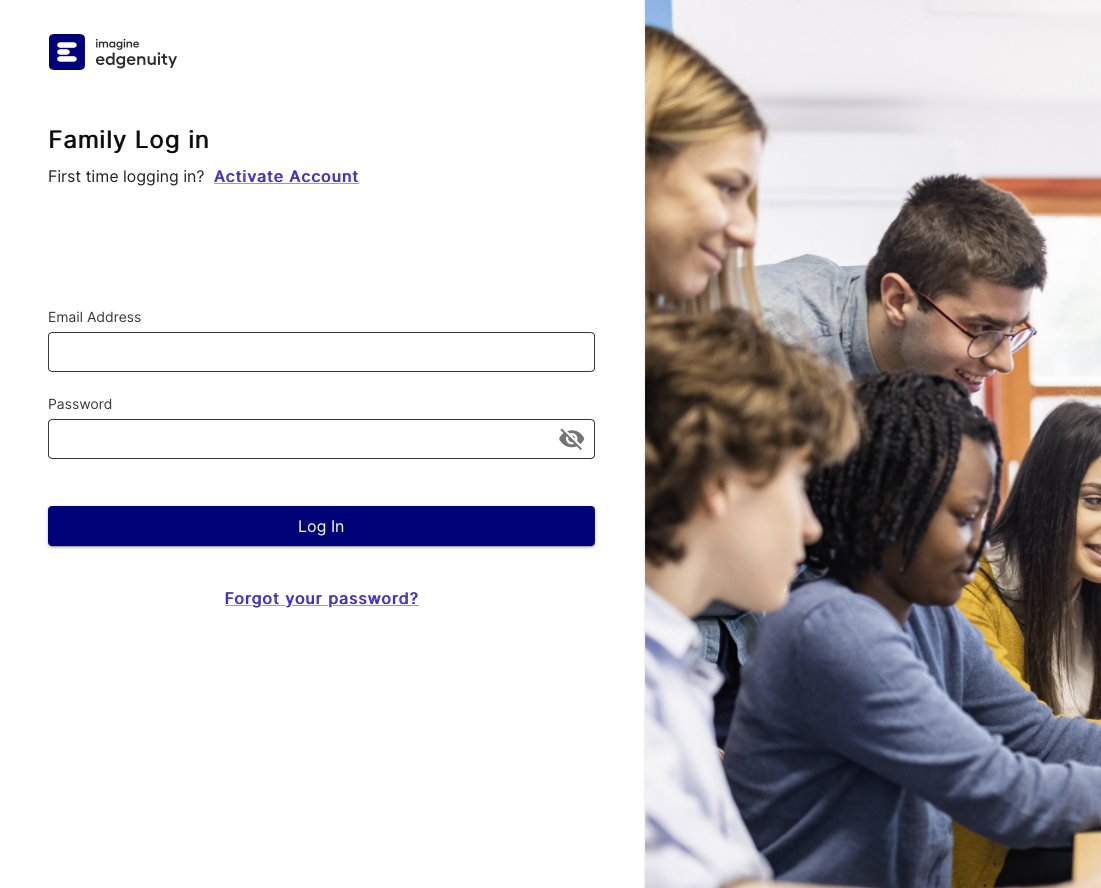The image features a split-screen capture divided into two distinct sections.

On the left side, there is a white background with text in black and purple fonts. At the top is a purple and white icon. Below the icon are the words "Imagine Ingenuity" in black. Following this, it reads "Family Login," "First time logging in?" and further instructs with "Activate Account" in purple. Two white input boxes with thin black borders are visible: one for an email address, which is blank, and another for a password, also blank, except for an eye icon with a slash through it, indicating hidden text. Under these boxes is a purple button with white text that says "Log In." Below this, in purple text, is a link reading "Forgot your password?"

On the right side of the screen, there is an image depicting a classroom or study session. The setting includes white walls and an orange wood-trimmed window. In the scene, a brown-haired man with glasses is leaning over the shoulder of a dark-haired female student, who is dressed in white and gold. Next to her, another student, an African-American woman with dreadlocks, is sitting and dressed in blue. Adjacent to her is another brown-haired student also dressed in blue. Further on the right side of the image is a female student with a large, prominent nose and blonde hair. The image is of good quality, clearly capturing the group of students engaged in their activity.

Overall, the image presents a functional login page and a vibrant educational scene, emphasizing the blend of digital accessibility and interactive learning.